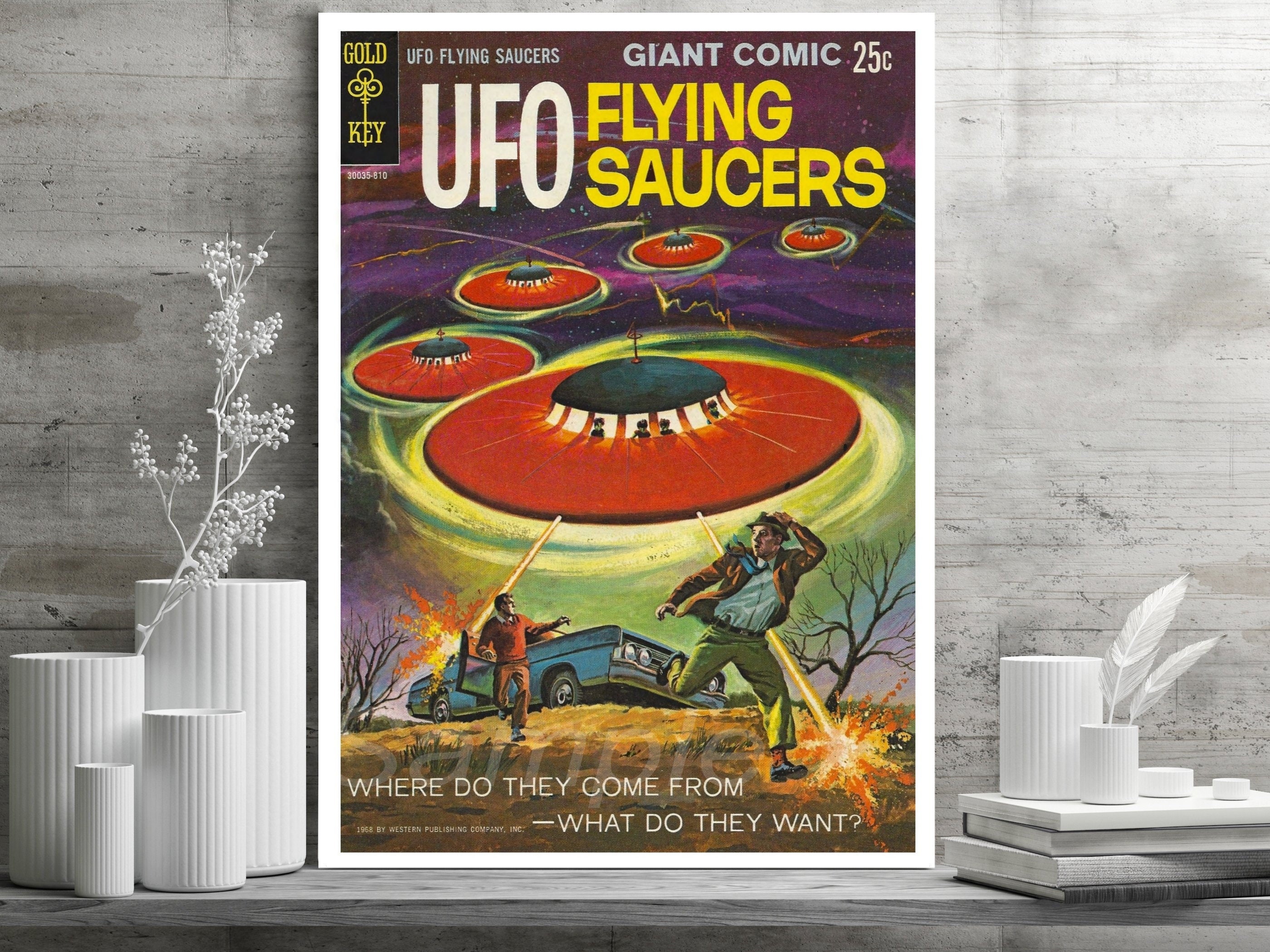The photograph, taken indoors, features a gray-washed wooden wall composed of horizontal slats and a matching narrow gray shelf at the bottom. On the left side of the shelf, there are four white cylindrical planters, with the leftmost one holding a single white-painted branch adorned with small beads or berries. On the right side of the shelf, there's a stack of four books with two matching white cylinders placed on top, one containing two white feathers. Central to the image is a large rectangular vintage comic poster, propped up against the wood wall. The poster, bordered in white, features a key in its upper left corner labeled "gold key" against a black background. The main title, "UFO Flying Saucers," appears in large white and gold print, advertising it as a "giant comic" costing 25 cents. The vivid illustration depicts five red flying saucers with black tops and visible alien silhouettes, hovering above a purple sky. The saucers shoot laser beams towards the ground, where two men flee from a blue car down a hill. The bottom of the poster asks, "Where do they come from? What do they want?"